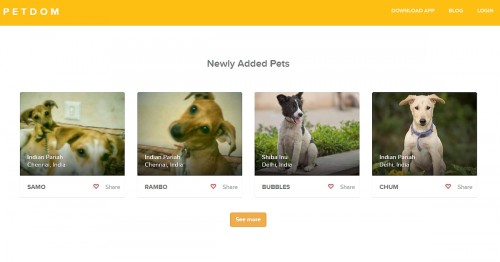The image, sourced from the Petdom website (P-E-T-D-O-M), features a yellow navigation bar at the top with the Petdom logo in white on the upper left corner. On the upper right corner, there are tabs labeled "Download App," "Blog," and "Login." Beneath the navigation bar, the background is white and displays the heading "Newly Added Pets" at the center. 

Below the heading, there are four pictures of pets:

1. The first picture shows two brown and white dogs named "Sammo." A share button is positioned to the right of this picture.
2. The second picture features a brown dog named "Rambo," with a share button to the right.
3. The third picture presents a black and white dog named "Bubbles," also with a share button to the right.
4. The final picture displays a white dog named "Chum." 

Below the series of pet images, there is a yellow-orange button labeled "Get Quote."